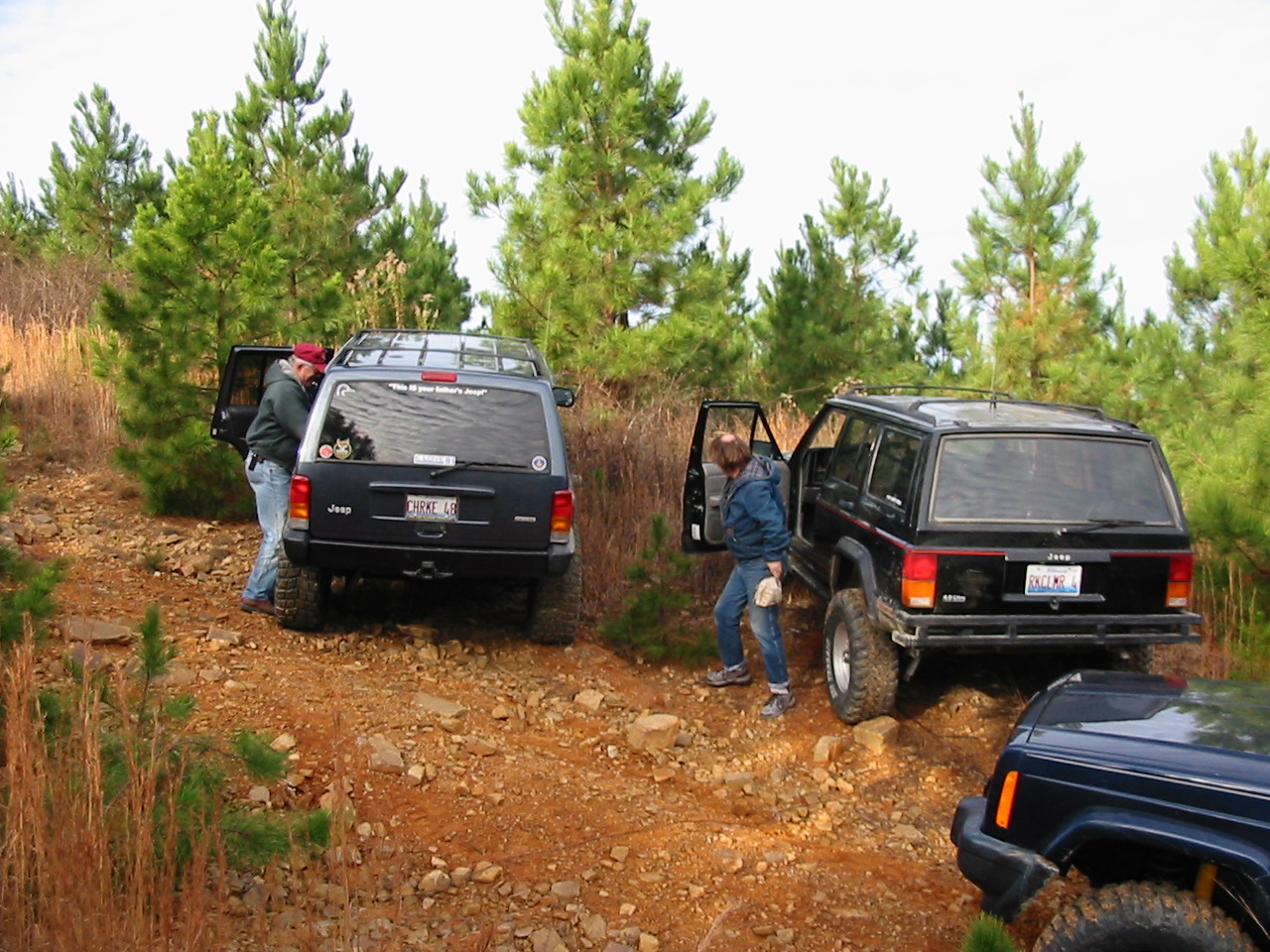In this captivating outdoor image, a dirt path meanders towards the top left, bordered by verdant green trees resembling short pine trees on the right. To the left, various small vegetation with brown stalks and green leaves suggest budding plants or baby trees. The path itself is a bright brown, earthy trail peppered with gray rocks. Along this road, three dark-colored, robust Jeep SUVs are parked. The vehicle on the bottom right is partially visible, only showing its front hood and tire. These vehicles boast distinct features: one is a dark navy blue, another is black, and a third is a sky blue. The Jeeps' brands are prominently displayed along with their red and orange tail lamps and white license plates with dark red text. Their mud-covered off-road tires, likely enhanced with lift kits, hint at rugged adventures. Doors on two of the Jeeps are open, with two men standing beside them - one in a blue jacket and jeans next to the right vehicle and another in a greenish hoodie or jacket and a red hat with jeans next to the left vehicle. The sky overhead is a typical sky blue, casting a natural light over this serene forested scene.